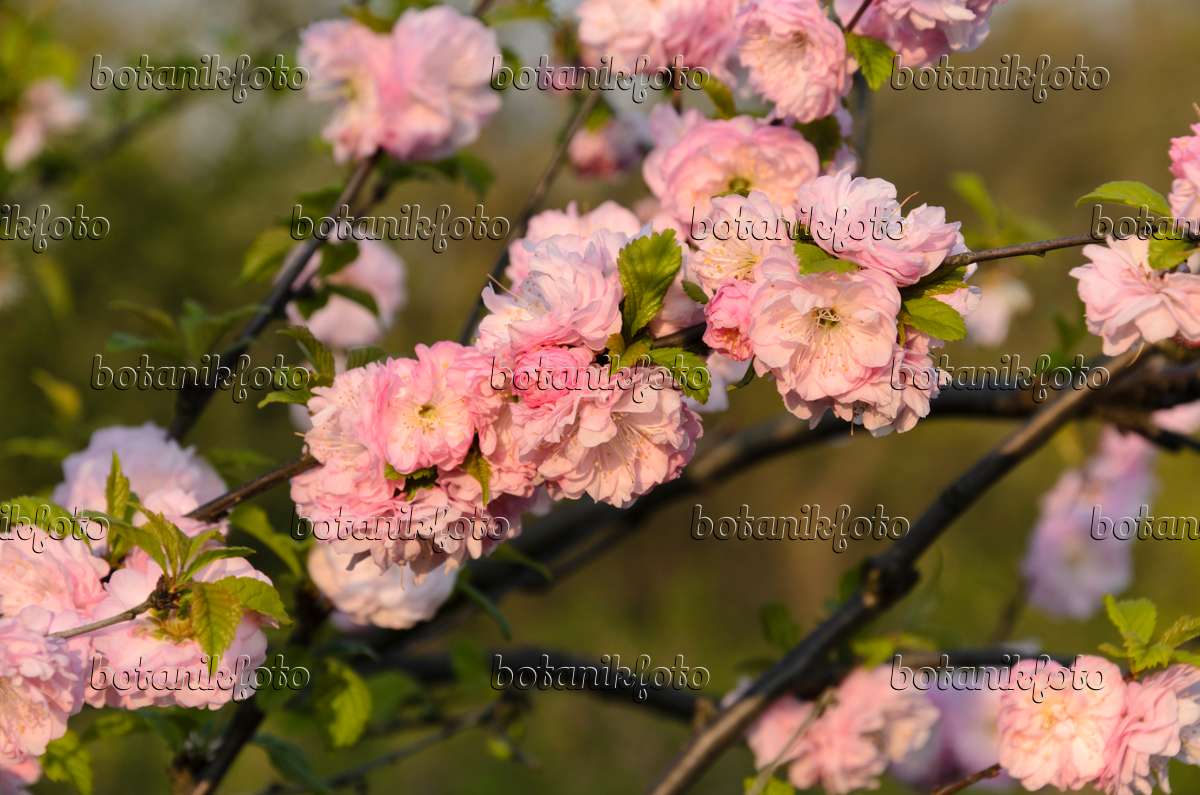This vibrant nature photo showcases a close-up of a plant adorned with clusters of light pink flowers. Each flower displays numerous interlocking petals with yellow stamens at their centers, while green leaves complement the colorful blossoms. The brown branches, though slightly blurred, slant from the lower left to the upper right of the image, providing a natural backdrop. The photo has an olive-ish background reminiscent of what one might see in nature. Repeated multiple times across the image, a watermark in lowercase reads "botanic foto."